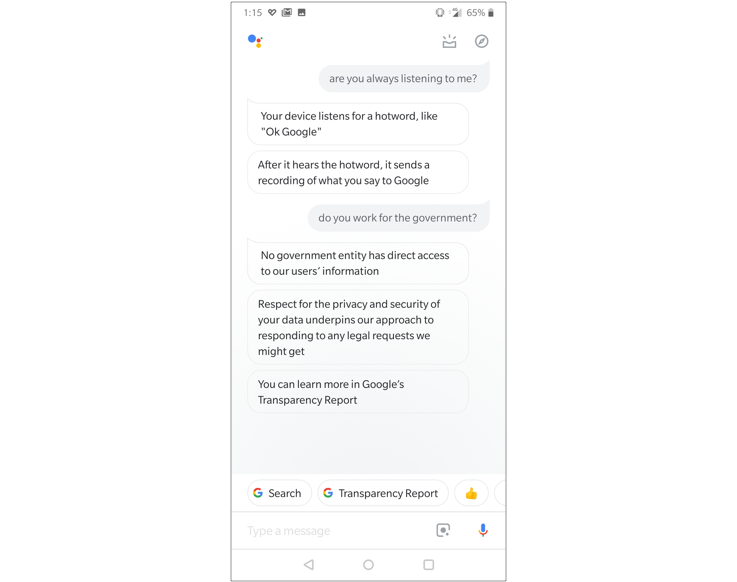Screenshot of a smartphone display with a clean white background. The top of the screen shows the time "1:15" in the top left corner and battery level at "65%" in the top right corner. Immediately below, there are three dots aligned to the left—one blue, one red, and one yellow.

A chat conversation is displayed with alternating gray and white chat bubbles. The first chat bubble appears from the right side in light gray, containing black text that reads, "Are you always listening to me?" The response appears in a white chat bubble with text explaining, "Your device listens for a hot word. After it hears the hot word, it sends a recording of what you say to Google."

Another light gray chat bubble from the right poses the question, "Do you work for the government?" This is followed by a detailed response in a white chat bubble: "No government entity has direct access to our users' information. The privacy and security of your data underpins our approach to responding to any legal requests we may receive. You can learn more in Google's Transparency Report."

At the bottom of the screen, there are navigation options labeled "Google Search" and "Google Transparency Report," accompanied by a thumbs-up icon.